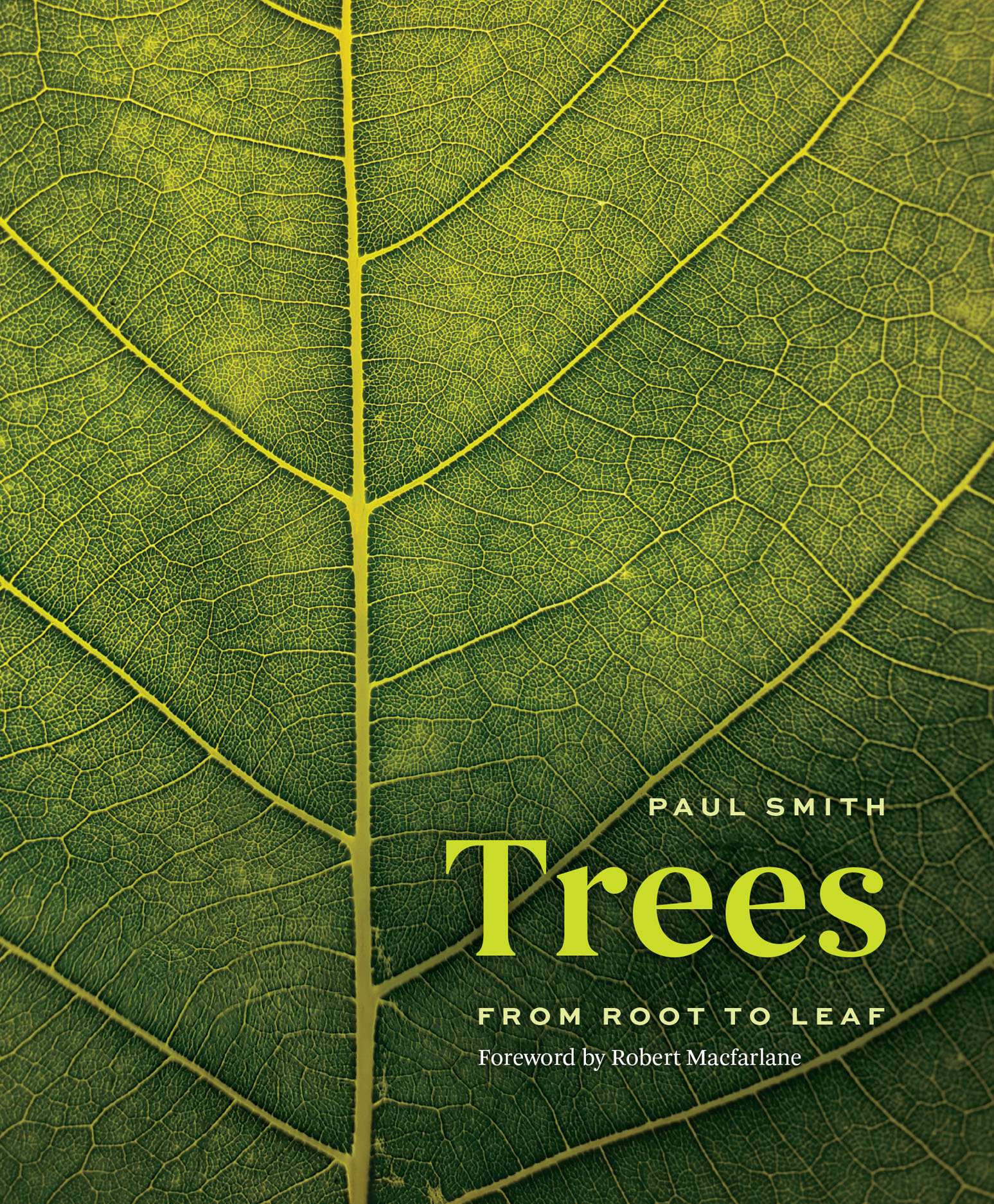The image features the cover of a coffee table book titled "Trees" by Paul Smith, with a foreword by Robert McFarlane. The cover photograph is an extreme close-up of the underside of a green leaf, filling the entire frame and showcasing its intricate yellow-green ribs and detailed veining. The title "Trees" is rendered in large, green font, while the subtitle "From Root to Leaf" and the author's name "Paul Smith" are presented in a plain white Arial-type font. All text is positioned in the lower right corner, allowing the magnified, almost microscopic detail of the leaf's cell structures to dominate the cover.